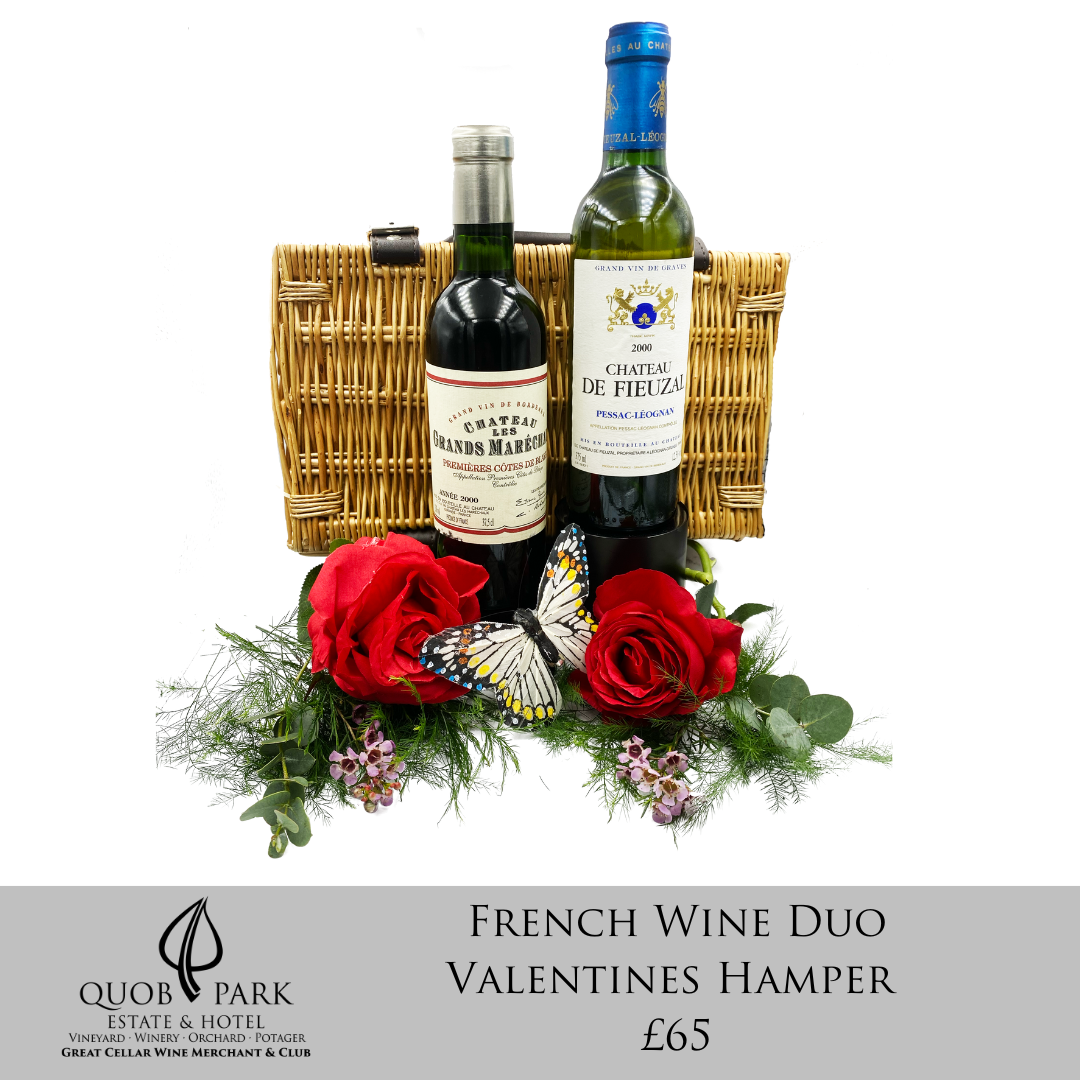The advertisement image displays a French wine duo Valentine's hamper priced at 65 pounds, as indicated by the gray band at the bottom. The banner also includes the logo of Crowe Park Estate and Hotel, Vineyards, Winery, Orchard, Great Cellar Wine Merchant, and Club. Above this text is a detailed product shot featuring a rectangular brown wicker picnic basket placed behind two bottles of French wine. The bottle on the right, taller and with a blue foil covering its cork and neck, is named Chateau Les Grands Morceaux, while the shorter, darker bottle on the left is labeled Chateau de Fuzon. In front of the bottles lies a charming floral arrangement, comprising two red roses, green sprigs, and small pinkish-purple flowers. A monarch butterfly with its wings spread is delicately perched among the roses, completing the elegant and romantic presentation.